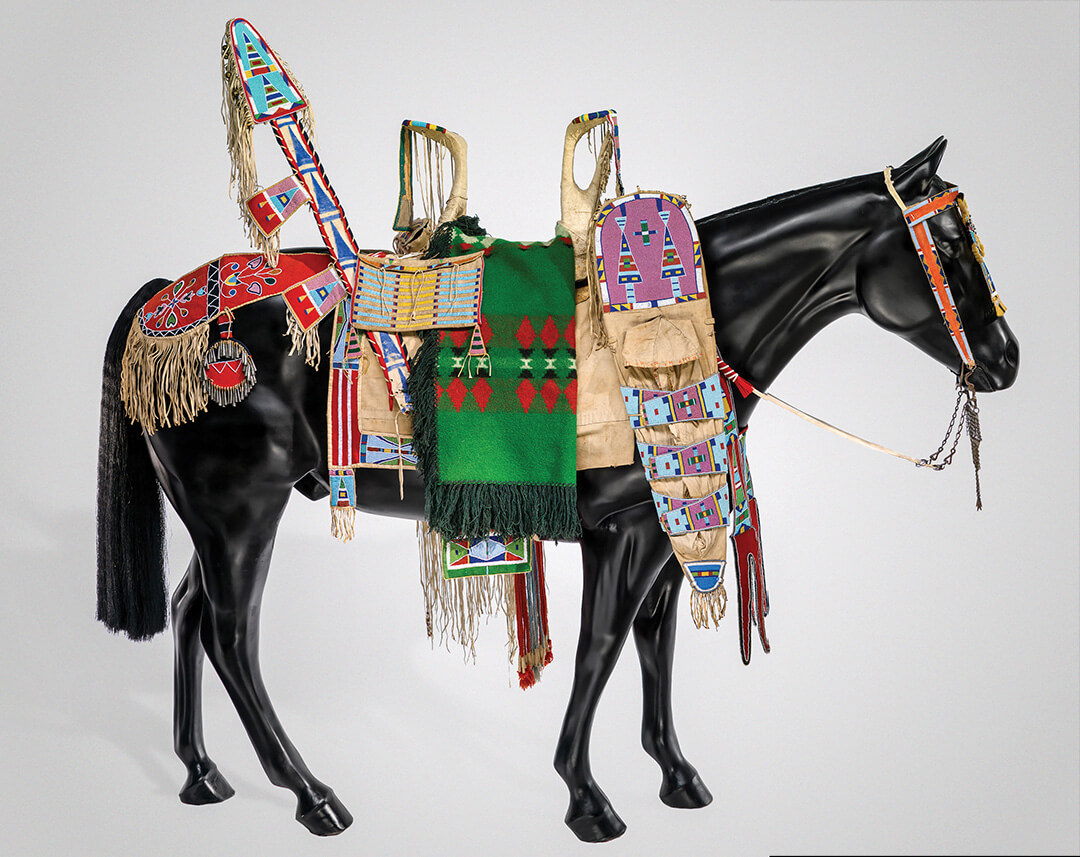The image depicts a prominently featured, solid black, lifelike horse model, likely crafted from plastic or fiberglass, centered against a plain white background. The horse is outfitted with an elaborate array of traditional-looking decorations, potentially inspired by Native American or Mongolian designs. This beautifully adorned horse faces to the right, showcasing a distinctive bridle in bright, contrasting colors of red, blue, and yellow. 

The saddle, an antique-looking piece in a light tan hue, is intricately carved and features long handles in both the front and back, indicative of classic, functional design. Draped over the saddle is a striking green blanket with red accents and fringes, creating a vivid visual contrast. Adjacent to the green blanket, on the side of the horse, hangs a long, oval-shaped shield decorated with geometric patterns in shades of purple and blue. 

The horse's hindquarters are covered with a red blanket that reaches down to its flank, adorned with floral designs, further enhancing the ornate presentation. Surrounding these principal elements are various other fringed and decorated pieces, each contributing to the overall intricate and indigenous aesthetic of this majestic horse sculpture.